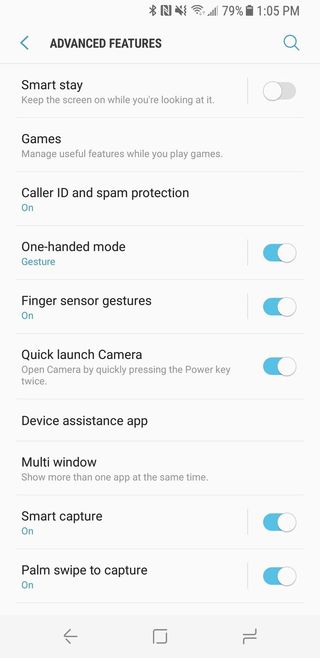This is an image capturing the settings screen of a smartphone, showcasing the "Advanced Features" menu. At the top of the screen, the "Smart Stay" option is visibly turned off, indicated by a gray slider positioned to the left. Further down, the settings for "Games", "Caller ID and Spam Protection" both display "On" statuses. The "One-handed Mode" setting is active, switched to gesture mode, with the slider positioned to the right, indicating it is turned on.

Continuing down the list, "Finger Sensor Gestures" is enabled, with the slider also in the on position. Similarly, "Quick Launch Camera" is active. The "Device Assistance App" and "Multi Window" options do not feature sliders. The "Smart Capture" setting shows it is on, with the corresponding slider to the right. Lastly, "Palm Swipe to Capture" is also turned on, evidenced by the slider positioned to the right.